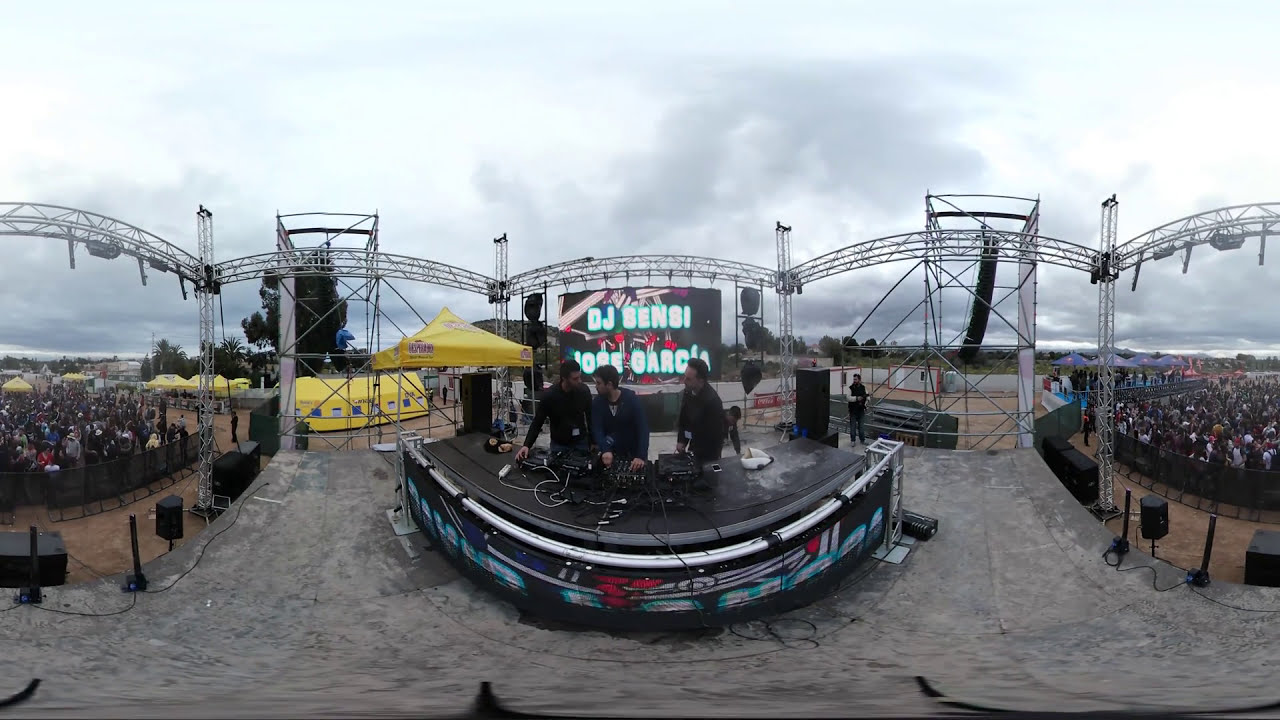The photograph features a 360-degree panoramic view of an outdoor event, capturing a stage where three DJs, all with dark short hair and dressed in dark clothing, are positioned behind a large arched semicircle table. The table appears distorted due to the panoramic effect and is adorned with various DJ equipment, including at least four black rectangular boxes with switches and wires spilling off the back and draping onto the gray cement-colored ground.

Above the DJs, there's a scaffolding setup with track lights and spotlights, while a large curved LED screen with bright letters, displaying text such as "DJ Sensi" and "Jose Garcia" against a patterned light background, forms the backdrop of the stage. The scene is framed by black fencing which encloses a dense audience standing shoulder to shoulder, eagerly facing the stage. On either side of the stage and back of the crowd, there are visible yellow and blue tents and canopies adding to the festive environment. The photo also captures additional details like black speakers positioned at the edge of the stage and a light banner or LCD screen running along the front of the DJ table, enhancing the overall visual appeal of the event.